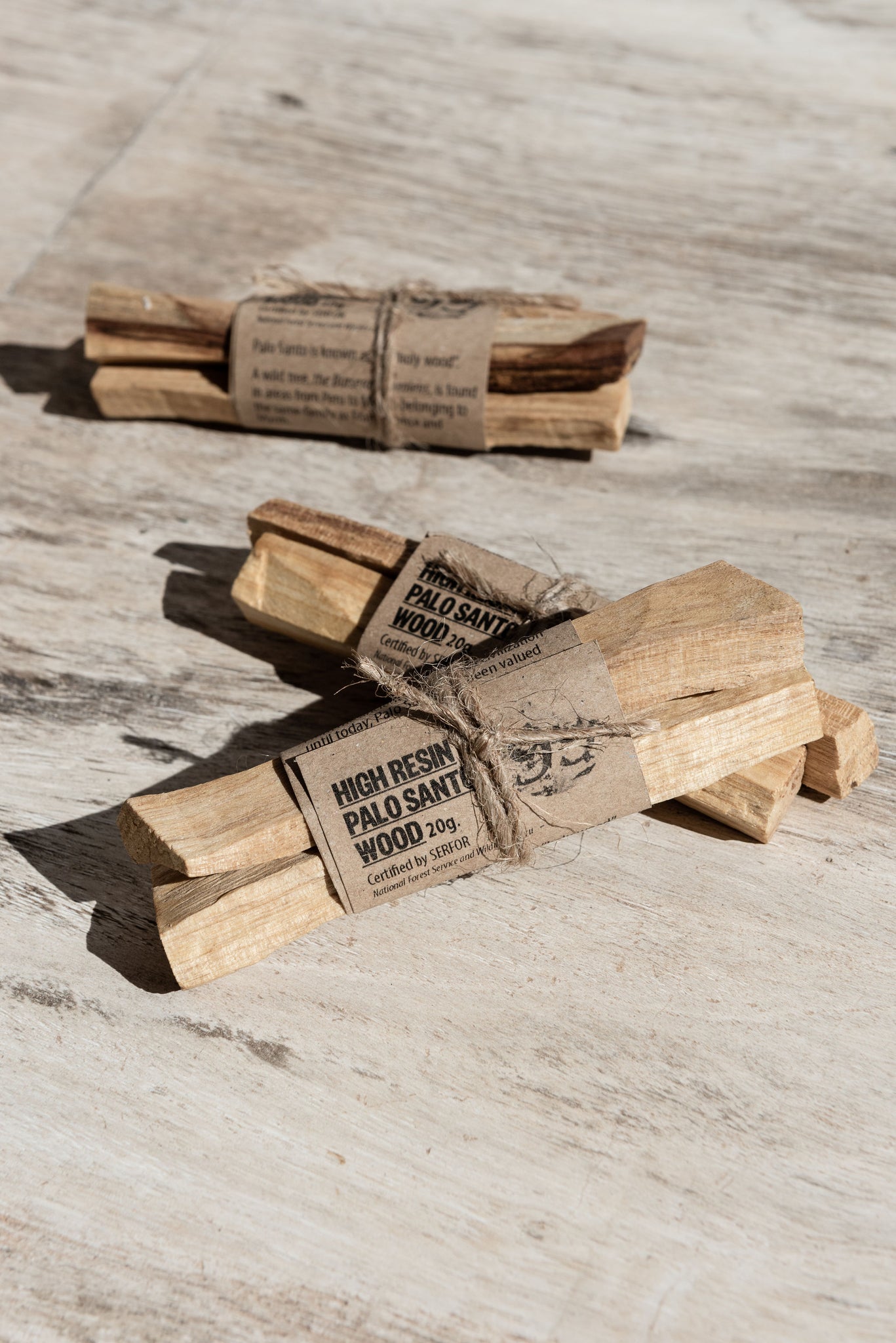This detailed color photograph captures three small bundles of Palo Santo wood arranged on a distinctive, light-colored wooden surface that features a pattern of white, light brown, and hints of dark gray. Each bundle is wrapped in a gray, cardboard-colored paper featuring black text that reads, "High Resin Palo Santo Wood, 20G, Certified by CERFOR, National Forest Service," though some of the text is hidden by twine. The bundles are neatly tied with rough, light brown string. In the foreground, two bundles are stacked; the one at the bottom is placed vertically while the one on top is diagonally oriented. A third bundle appears out of focus in the background, adding depth to the composition. The Palo Santo wood sticks are pale in color, complementing the rustic wrapping and tying materials.